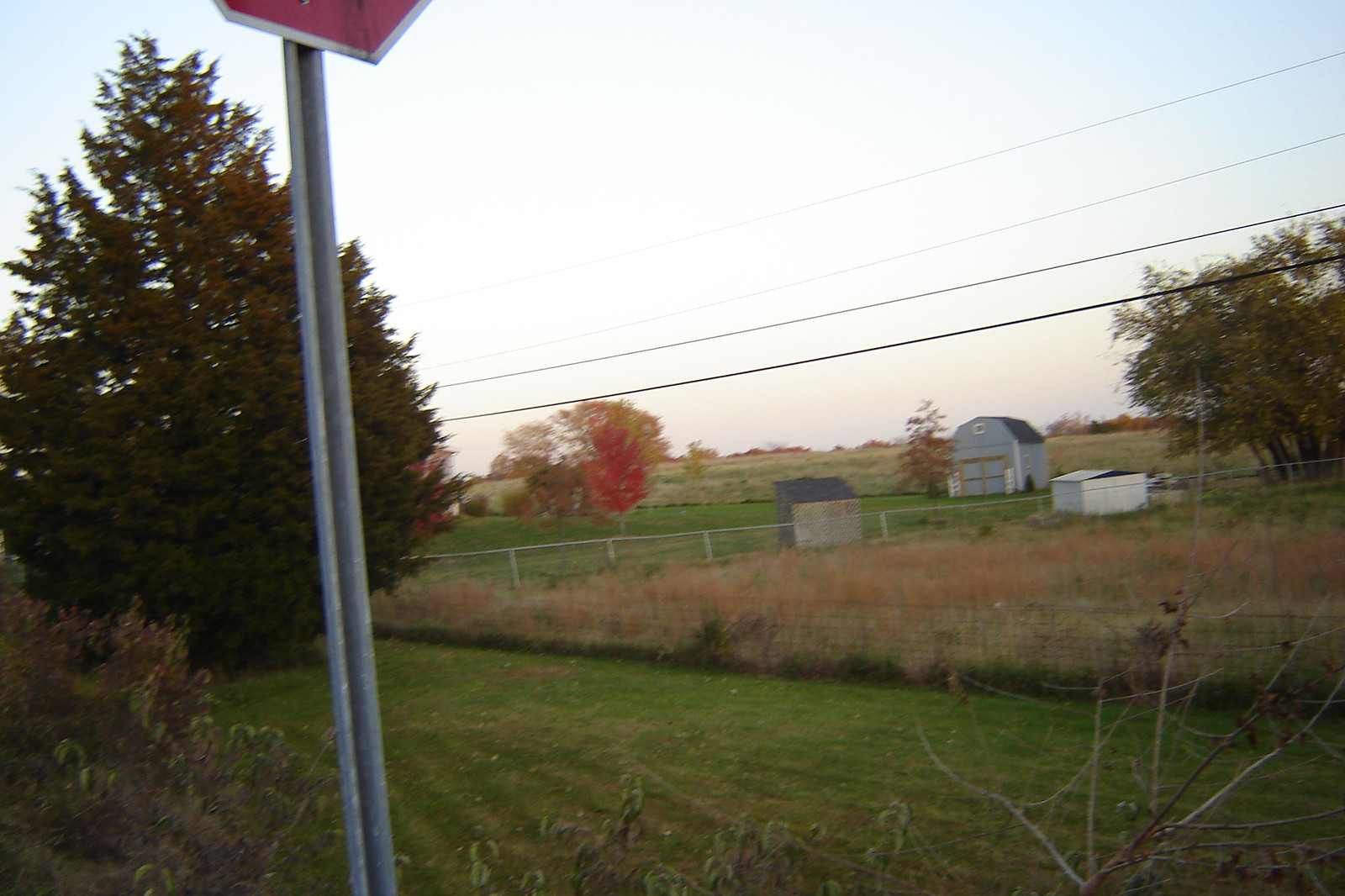The photograph captures a secluded farm property featuring a scenic grass meadow bisected by a gray chain link fence. To the right of the meadow, there's a sprawling field of brown plants, possibly wheat. The image also shows a series of sheds and small buildings in varying colors: a light blue, small home-like barn shed, a smaller white shed, and a light brown and black shed. Trees, in beautiful fall colors of orangeish-red and green, dot the landscape, suggesting it's autumn. Prominent in the left foreground, there's a gray metal pole topped by a stop sign. The blue sky above is interrupted by telephone wires running horizontally across the scene, further adding to the rustic visual. Bushes or underbrush are visible at the bottom corners of the image, enhancing the natural, untouched feel of the area.